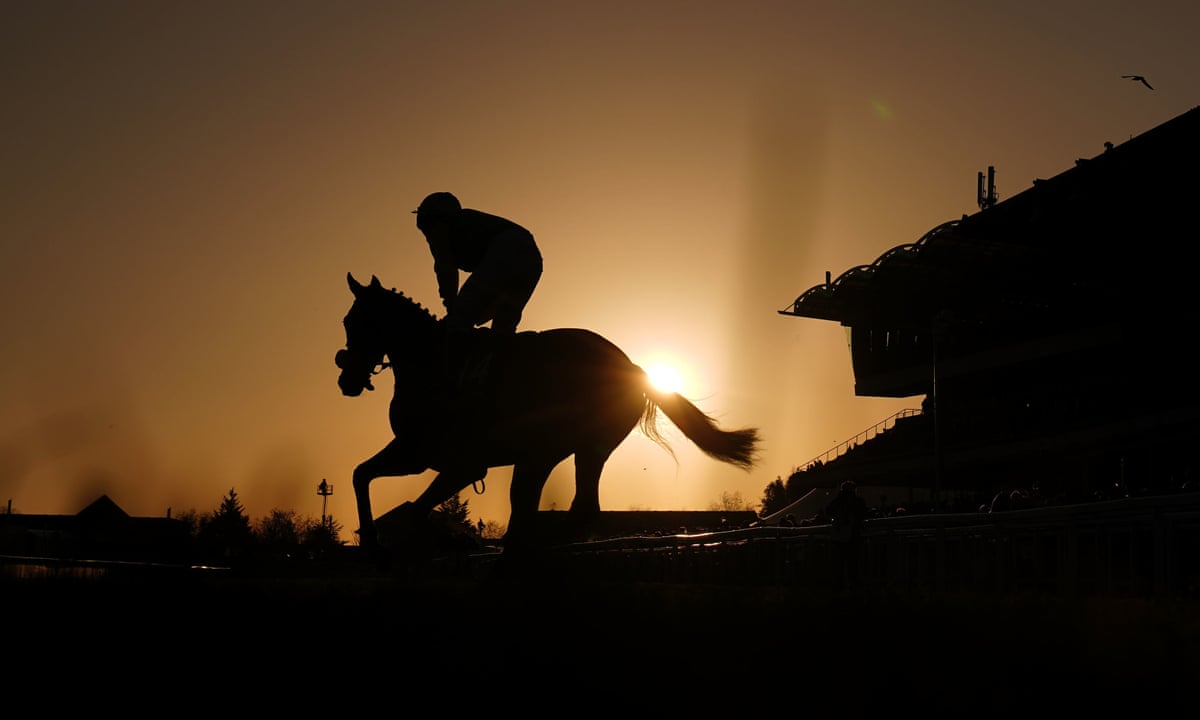This captivating image captures the serene yet dynamic moment of a jockey riding a galloping horse at either sunrise or sunset. The horse, moving swiftly towards the left of the frame, is highlighted by the sun appearing just above its back leg and tail, casting a radiant glow through its blowing braided mane and full bridling gear. The jockey is positioned in a standing stance, encapsulating an action shot amidst a setting bathed in hues of dark brown and pale coffee. The lower third of the image is enveloped in darkness, with just the edges of structures beginning to emerge in the early light. To the right, the silhouette of what seems to be a racecourse building stands, with a bird soaring above it. The entire scene, with its black and copper tones, creates a stark contrast, rendering all details as striking silhouettes against the brightening sky. Outlines of trees, bushes, and a street lamp subtly fade into the background, adding depth to this mesmerizing equestrian scene.